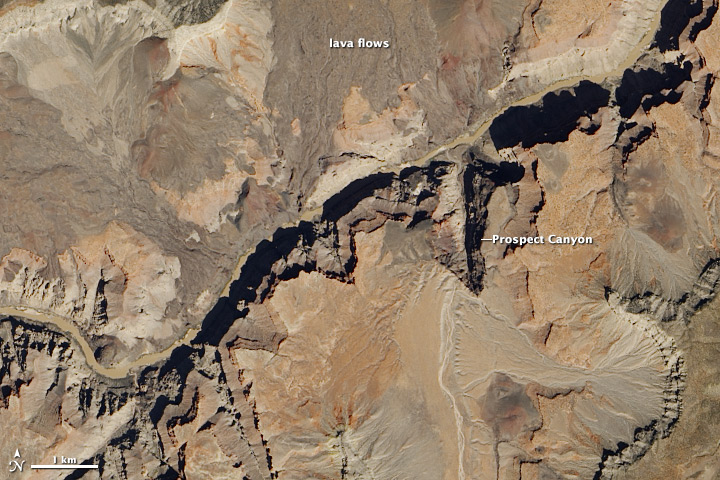This high-resolution aerial or satellite image depicts a desolate, rugged landscape marked by various shades of brown, gray, and tan, capturing the textured surface of mountainous and canyon-like terrain. A prominent, steep ridge runs diagonally from the lower left to the upper right, casting dark shadows that accentuate its sharpness. The top section of the image is labeled "Lava Flows" in white letters, indicating the area likely features remnants of ancient volcanic activity. Below this ridge, towards the center-right of the image, "Prospect Canyon" is denoted, suggesting a specific geological interest. In the lower left corner, a scale bar labeled "1 kilometer" provides a reference for the area's extent alongside an arrow pointing north (N). The image lacks visible vegetation, emphasizing a barren, rocky expanse.